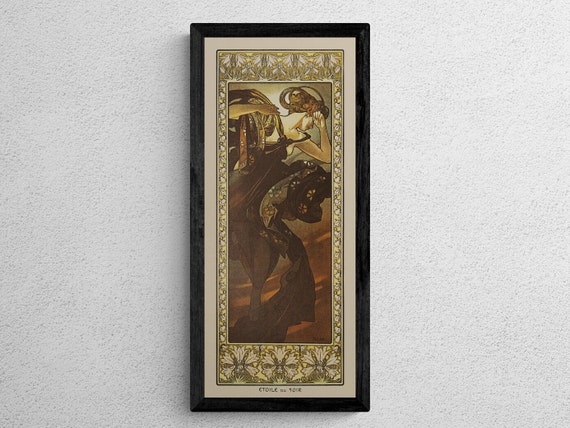The image depicts a tall, vertically oriented, rectangular painting mounted on a light gray or light blue wall with a hint of popcorn texture. The painting is encased in a black, beveled frame, devoid of any intricate designs. Inside the main frame is a secondary trim with a mixture of gray, white, light tan, and gold borders, some of which bear decorative designs that extend to the top and bottom as well as thin strips along the sides.

The focal point of the painting is a woman who embodies an art deco style, reflective of the 1920s. Her left arm is raised, and her head is turned to face left, suggesting a sense of distress or contemplation. She has her brown hair pulled back and is clad in an elaborate, frilly black gown with a long train. The gown seems to have dusty brown and red hues with small floral patterns. She holds an indistinct object in her right hand. The background features a reddish sky that might depict her riding a black horse, enhancing the dramatic ambiance of the scene. The overall colors of the painting are brown, gold, and cream, contributing to its vintage aesthetic.